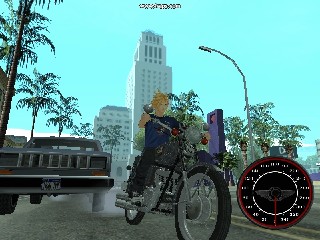In this video game screenshot, a young blonde male character wearing a blue t-shirt and black pants is riding a thin motorcycle that resembles a bicycle. The motorcycle’s large front wheel with silver spokes is prominent. To the left of the motorcycle is the front end of a car, with smoke around its left tire, likely from the motorcycle's motion. A black speedometer with a red border is displayed in the bottom right corner of the image. The scene is set against a backdrop featuring a tall white building in the center, with a smaller mid-rise building next to it. The background also includes tall streetlights and palm trees on both sides, giving an LA-like atmosphere. At the top of the image, there is a foreign language phrase that is too small to read clearly.